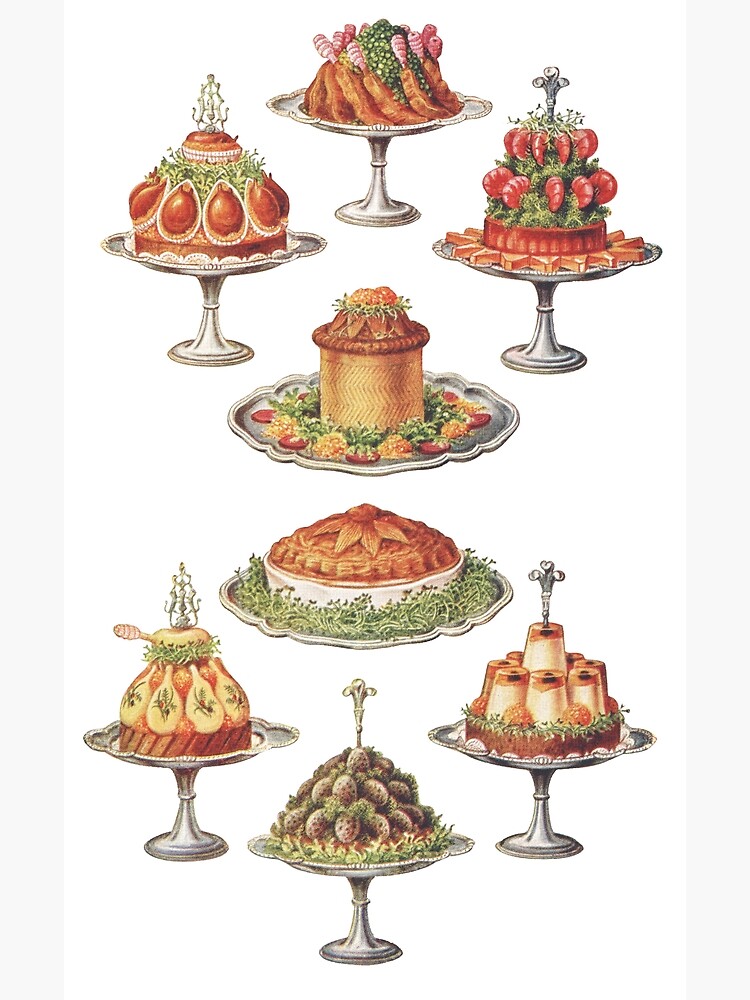The image depicts a series of elevated silver and gray trays showcasing an array of intricate, holiday-themed dessert and entree illustrations. The background is a solid white, accentuating the colorful food items. At the top, a dish resembling a strip of meat with pink tips rests atop a mound of peas. Below it lies an oval-shaped meat adorned with white pearls, seated on a cake surrounded by lettuce. The two trays in the middle are flat, displaying a cupcake topped with a silver emblem, and an arrangement of shrimp and greens on a cake with silver detailing. Among the illustrations are a tall cylinder featuring fish, sliced pepperoni, and an orange substance; a star-designed cake; a drumstick-shaped white meat with embedded herbs; meatballs or potatoes among greens; and a jello dessert in white and orange hues. Most items are enhanced with green vegetables or floral garnishes, contributing to the festive and lavish nature of the display.